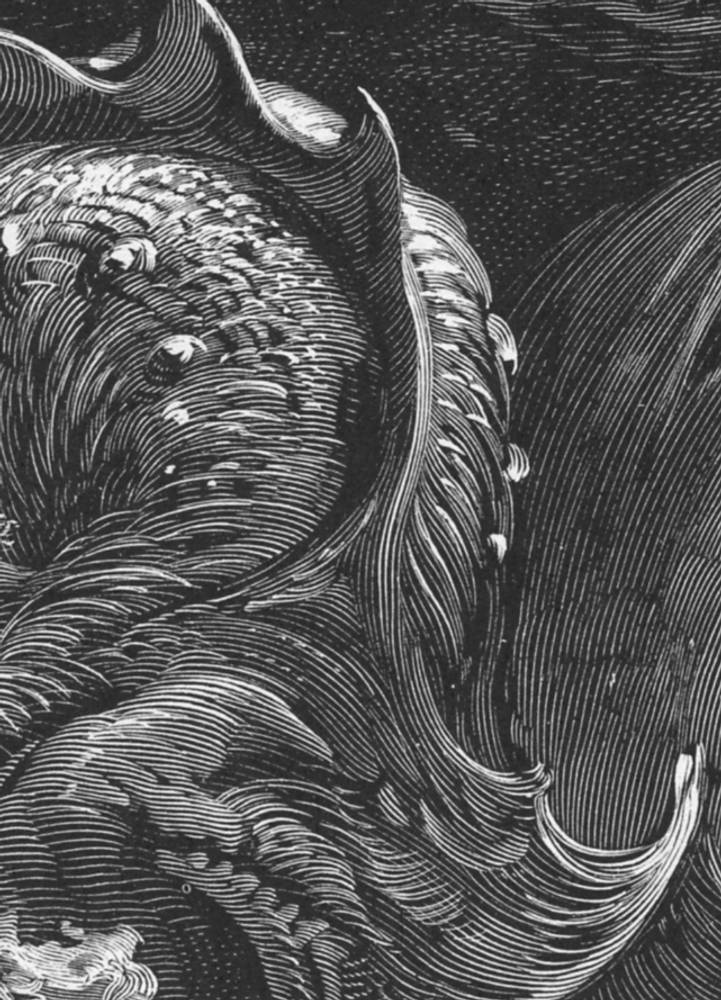This is a detailed close-up of a black-and-white drawing, resembling a dragon's spine. The monochromatic image, possibly created with black pen strokes or pencils, shows intricate, swooping lines that hint at motion. The central focus is a curved, scaly structure starting from the upper left corner, descending vertically towards the center and bottom of the image. This structure features a ridge or fin-like formation with pointed spikes running along the top, suggesting a dragon-like appearance. The grayscale tones and dense line work create a visually dynamic and textured scene, possibly reminiscent of a woodcut or an illustration from a book or magazine.